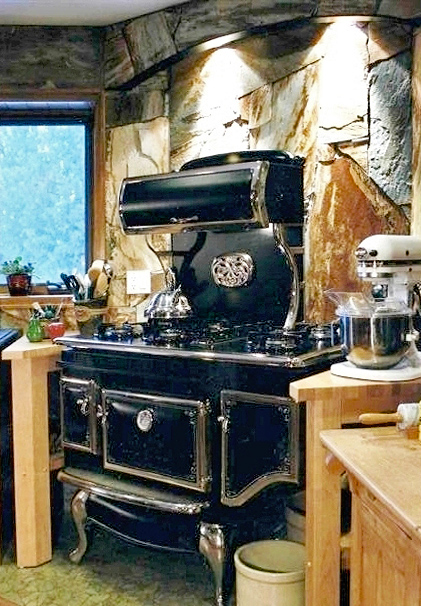This photograph captures a rustic, antique kitchen centered around an old-fashioned, black stove with metallic silver trimmings and gold-tone legs and drawers. The stove, reminiscent of the 1920s or 30s, stands proudly on four decorative legs and is nestled into a stone wall made from slate and limestone. It features multiple doors for wood and ash management, a gas range on top, and is illuminated by recessed lighting from the hood above.

To the right of the stove is a modern, white stand mixer with a silver bowl, contrasting with the vintage aesthetic. On the wooden countertops surrounding the stove, various kitchen utensils, including a rolling pin and condiments, add to the homely atmosphere. A silver kettle sits on the stovetop, further enhancing the nostalgic feel.

The kitchen boasts pine wood cabinets with open legs, and the floor is paved with green granite or marble, giving it a polished look. Natural light floods in through windows on either side, reflecting off green foliage and a few potted plants, creating a serene and timeless setting.